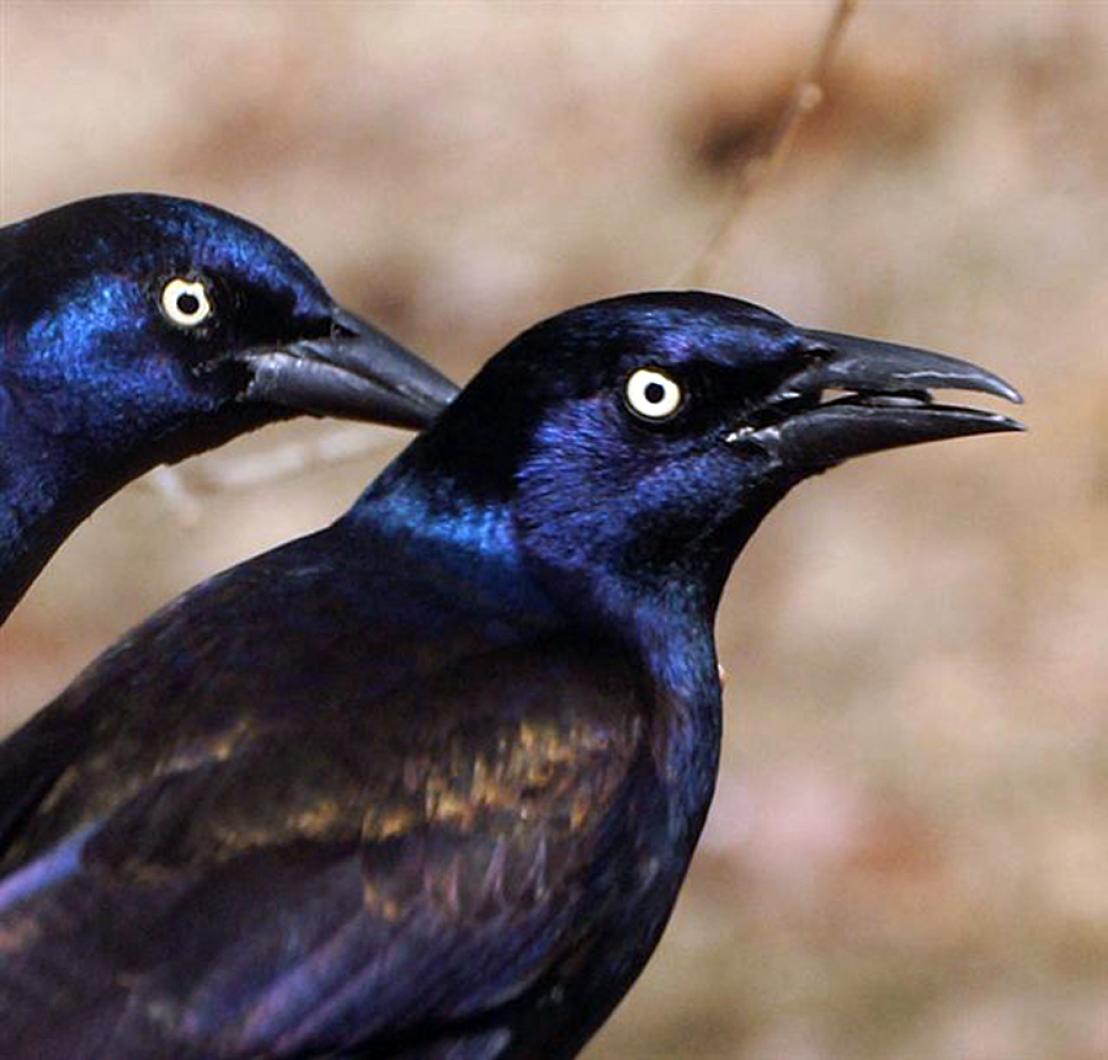The image is a close-up, color photograph of two black-feathered birds, likely crows or ravens, facing to the right. Their plumage is predominantly black with deep purple and dark blue accents, especially noticeable on their wings and around their head and neck. They have bright white eyes with black pupils and black beaks. The bird in the front has its beak slightly open, revealing a black tongue, and a faint yellow crust can be seen at the corner of its beak. The background is blurred, showcasing natural hues of beige and white with a subtle upward-curving stick, suggesting a ground setting.